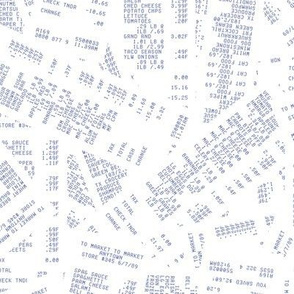This is a detailed black and white illustrative graphic designed to resemble multiple grocery receipts piled and fanned out on top of each other. The receipts, with black text on a white background, display typical elements like item names, prices on the right, and terms such as "tax," "total," "cash," and "change." The text includes a visible reference to "to market, to market" and "any town" at the top of one receipt, followed by store details. Despite appearing realistic, these are mock receipts created digitally, likely intended for use on shopping or money-saving sites. The image, with its vertically and horizontally oriented receipts, forms a cohesive wallpaper-like design without any borders, emphasizing the repetitive nature of the receipts and their contents.